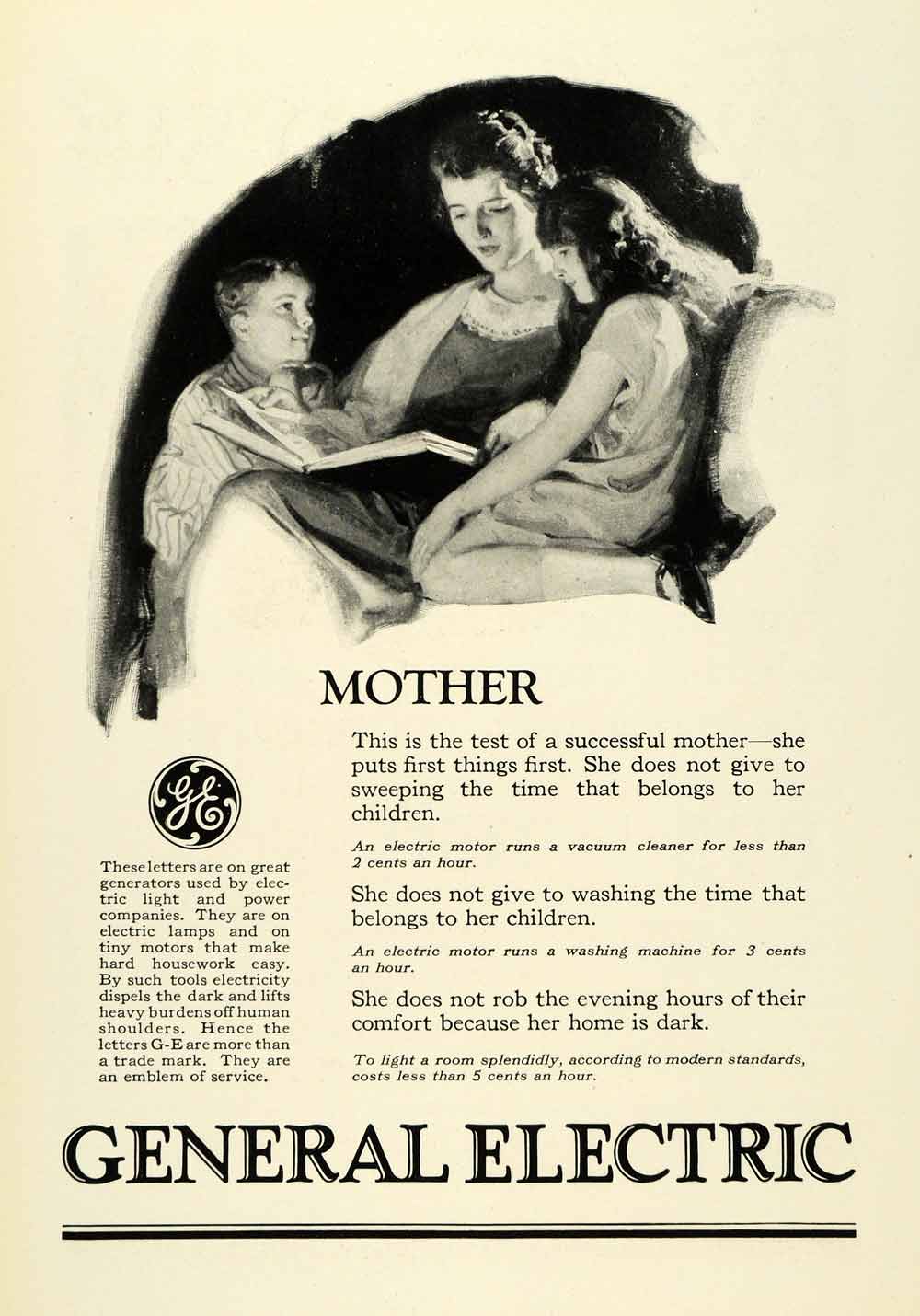This full-page vertically aligned rectangular advertisement, set against a beige paper background, prominently features a nostalgic black-and-white illustration of a mother with her two children, a boy on the left and a girl on the right, all gathered intimately around a book she is reading from. Beneath this touching family portrait, in bold black letters, the word "MOTHER" stands out as a header to a heartfelt message celebrating maternal devotion. The message, justified in alignment, emphasizes the virtues of a successful mother, stating: "This is the test of a successful mother. She puts first things first. She does not give to sweeping the time that belongs to her children. An electric motor runs a vacuum cleaner for less than two cents an hour. She does not give to washing the time that belongs to her children. An electric motor runs a washing machine for three cents an hour. She does not rob the evening hours of their comfort because her home is dark. To light a room splendidly according to modern standards costs less than five cents an hour." Adjacent to this text, on the left side, is the iconic GE logo, under which a brief paragraph elaborates on the brand's representation. The advertisement is rounded off with "GENERAL ELECTRIC" in large, bold capital letters centered at the bottom, underscoring the timeless value of modern conveniences in supporting dedicated mothers.